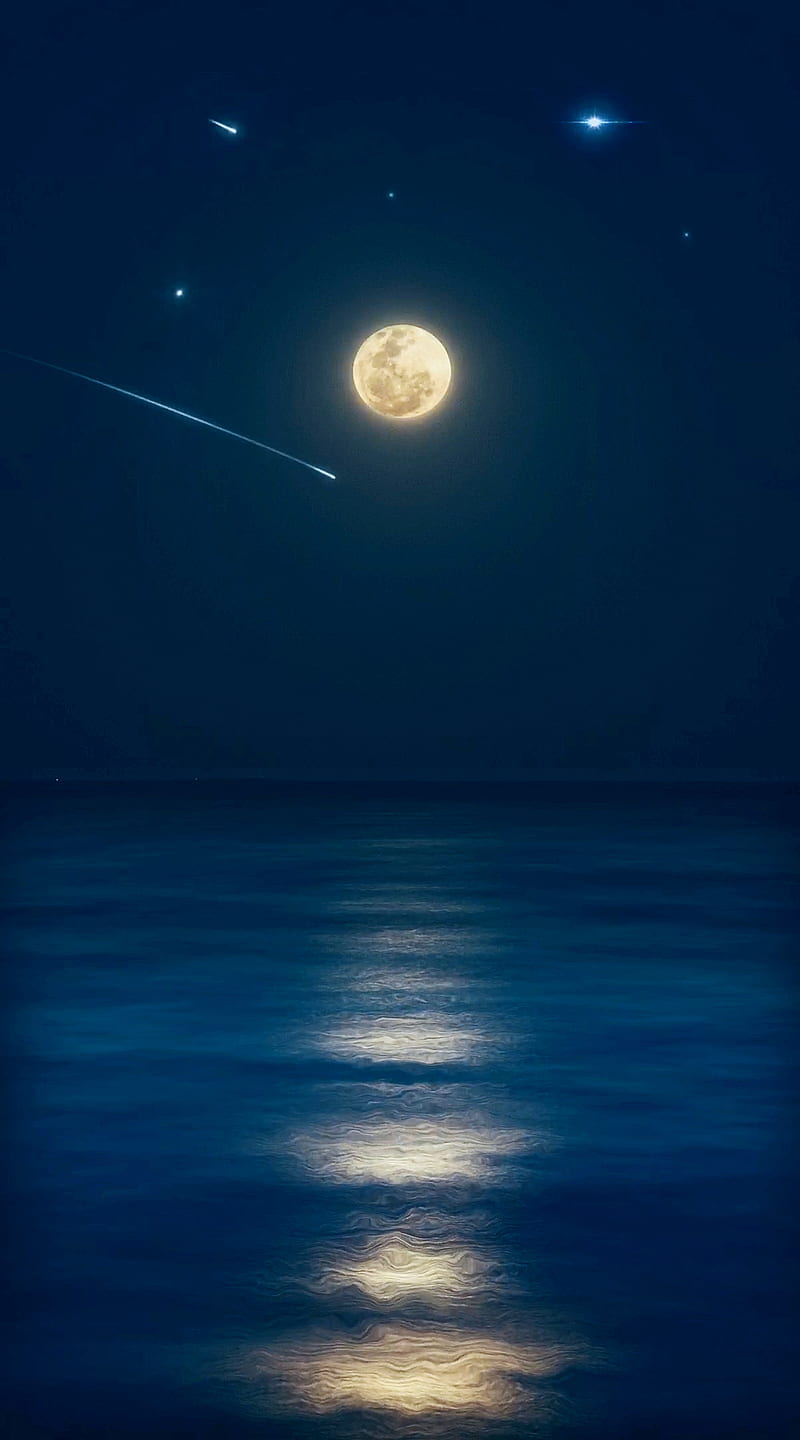The image is a detailed, surreal painting or drawing depicting a serene night scene over an ocean. Dominating the upper center of the vertically oriented rectangular canvas is a luminous full moon, casting a soft glow against the backdrop of a dark blue sky that graduates to black at the corners. The moon, with subtle brown spots on its left side and a halo around it, reflects in the calm ocean below, creating a row of five ghostly, successive moon images on the water’s surface. The horizon line, where the ocean meets the sky, bisects the image horizontally in the middle. In the sky, several stars of varying brightness are scattered, adding to the celestial ambiance. A prominent comet streaks diagonally from the upper left to the lower right, just beneath the moon, while another meteor with a shorter tail is visible at the top. The water beneath the moon reveals a hint of waves and motion, painted in shades of blue, purple, and black, enhancing the nocturnal beauty of the scene.